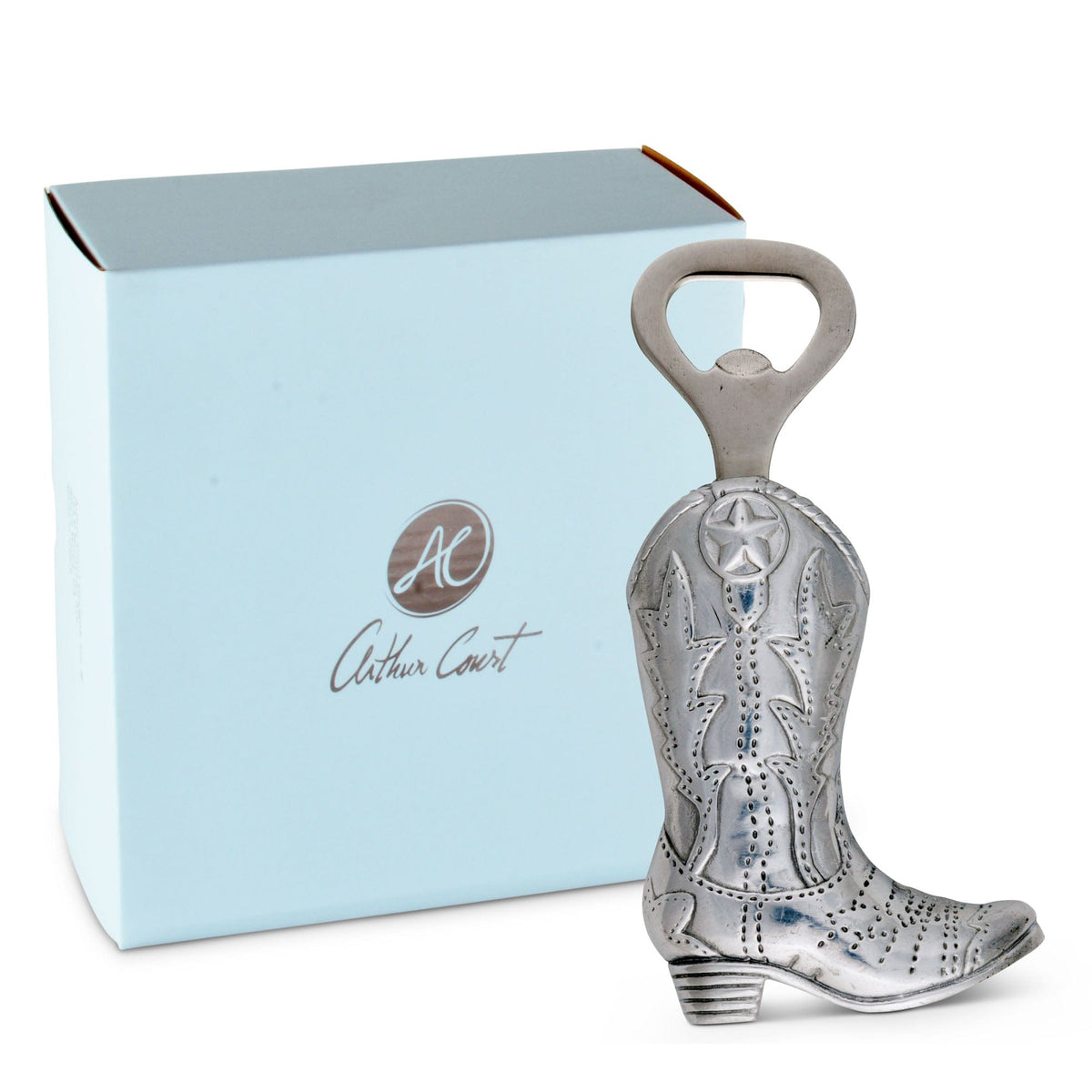The image showcases a product photo of a uniquely designed bottle opener. The handle of the opener is shaped like a detailed metallic cowboy boot, with intricate patterns, stitch marks, and a star design adorning the upper portion. The boot, which features a rounded toe and heel, adds a decorative touch to the otherwise functional tool. The bottle opener mechanism is positioned at the top of the boot. 

Behind the boot, there is a light blue box with closed flaps. The box displays a circular brown logo with the initials "AC." Below the logo, the name "Arthur Court" is written in a signature-style font. The background of the image is white, making the silver boot and the blue box stand out prominently. A hint of blue on the silver boot ties the elements of the image together, emphasizing the product's aesthetic appeal.